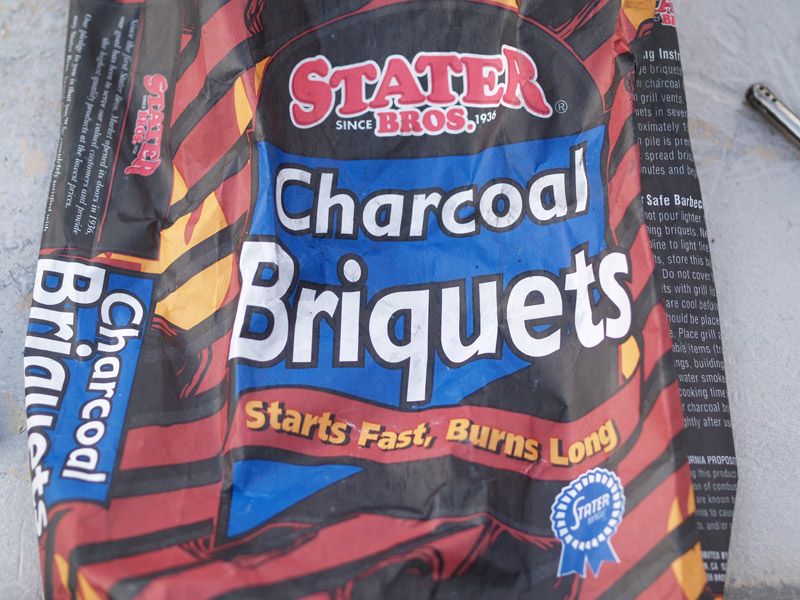This image depicts a partially empty bag of Stater Bros charcoal briquettes. The visually striking bag features prominent red stripes and displays the Stater Bros logo, a black oval with the text "Since 1934." Beneath the logo, a blue banner with white letters reads "Charcoal Briquettes," bordered in black. Lower on the bag, a statement within a red bar declares, "Starts Fast, Burns Long," accompanied by a blue ribbon indicating "Starter." The bag's design also includes elements like yellow flames and additional product information on the sides, although some text is obscured by the way the bag is folded. The bag is positioned against a table, with a fire lighter or starter barely visible in the top right corner, suggesting readiness for grilling.